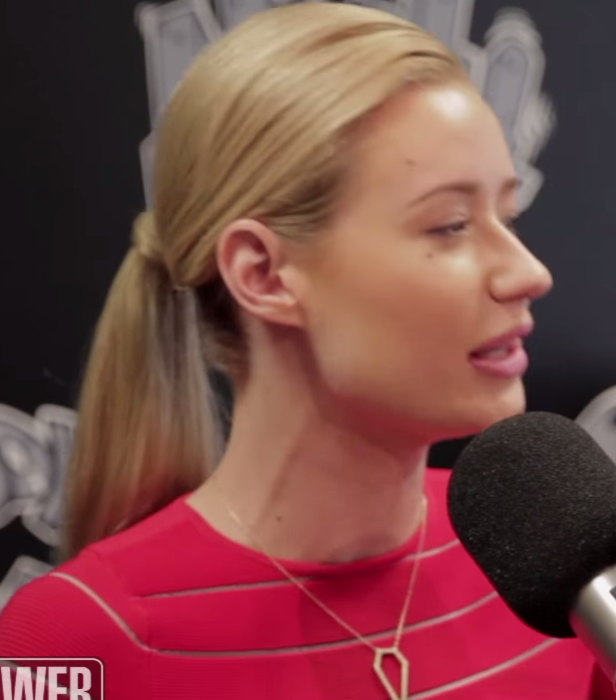Here's a detailed and cleaned-up caption for the image:

"Featured in the image is a likely actress or singer with long, flowing blonde hair styled in a ponytail, possibly Iggy Azalea. She is dressed in a striking red top and adorned with a delicate necklace that sports a coffin-shaped pendant. Notably, she is not wearing any earrings. The backdrop behind her is an all-black display, slightly blurry, making it difficult to discern its details. In the bottom left corner, there is the word 'web' accompanied by an indistinct logo. Also visible in the foreground is a microphone with a sizable cap."